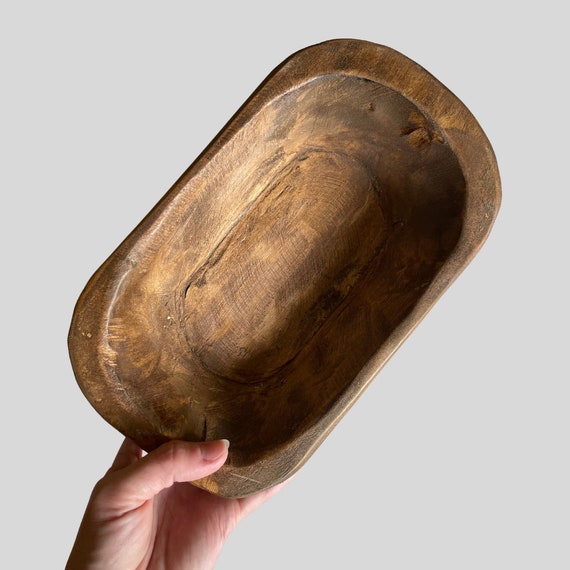In the photograph, a hand, likely belonging to a woman with a neatly manicured white thumbnail, is holding up an oblong wooden bowl against a featureless light gray background. The bowl is an elongated rectangle with rounded corners, showcasing a smooth texture and a striking wood grain in various shades of light and dark brown. The bowl's design features a narrower base that gradually curves up to a broader rim, giving it a distinct indent in the middle. Only the left hand, placed in the lower left-hand corner of the frame, is visible, holding the bowl at an angle that emphasizes both the craftsmanship and the natural beauty of the wood.